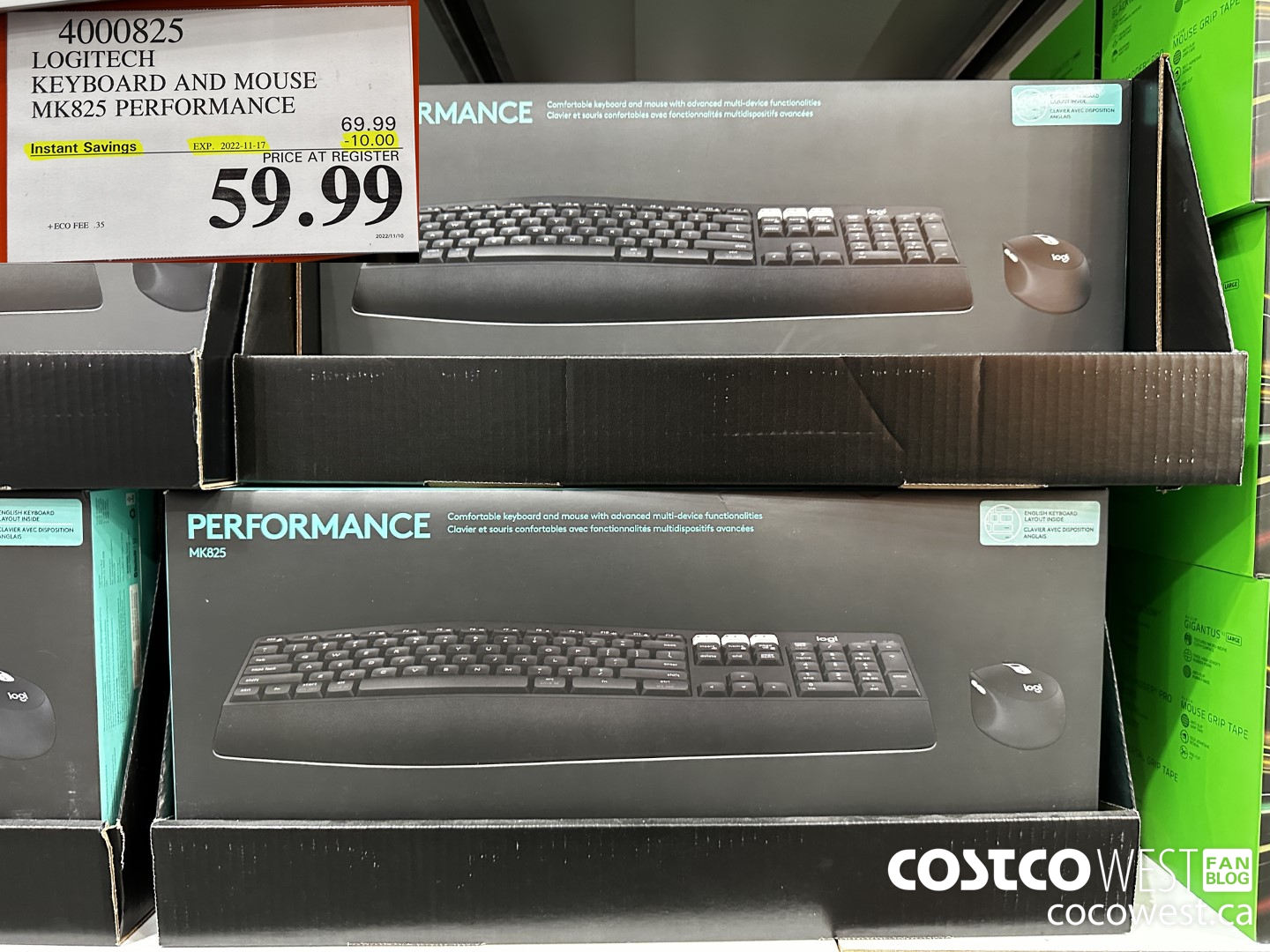A promotional image from the Canadian Costco West FanBlog (CocoaWest.ca) showcases a boxed wireless keyboard and mouse combo by Logitech, model MK825 Performance. In the foreground, a sticker prominently displays product details: item number 400082, original price of CAD $69.99, and a discounted price of CAD $59.99, highlighted in yellow to indicate instant savings. The expiration date of the offer, 2022-11-17, and a note indicating a saving of CAD $10.00, are also highlighted in yellow. Behind the sticker, several boxes of the keyboard and mouse combo are stacked, with one box open to show the contents inside. The box design features bold blue text stating "Performance" and "Comfortable Keyboard and Mouse Advanced Multi-Device Functionality," with the same text provided in French below.